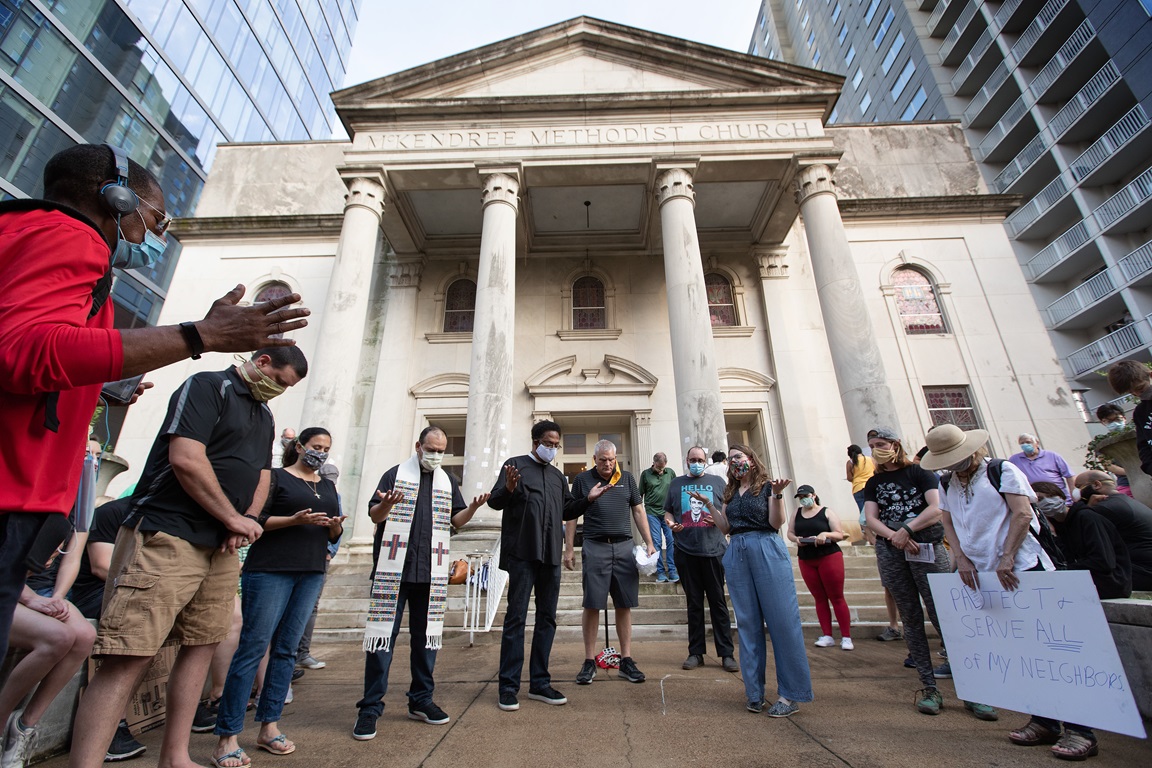In this photograph, a diverse group of about ten individuals is gathered outside the McKendree Methodist Church, a large, classical marble building distinguished by its tall portico, four white stone columns, and a peaked stone roof. The scene is set in a metropolitan area, indicated by the tall city buildings visible on either side of the church. The participants form a semicircle and appear to be praying, with their heads bowed, some having their arms outstretched. Most people, adorned in casual attire including jeans, leggings, and sweatpants, are wearing face masks, suggesting this event occurred during the COVID-19 pandemic. A notable figure, likely a priest, stands out in black clothing and a white stole marked with crosses. Additionally, a woman on the far right, distinguished by a straw hat, holds a sign that reads, "Protect and serve all of my neighbors." The mixture of religious solemnity and the presence of protest signs hints at a prayer service intertwined with a demonstration for a social cause.